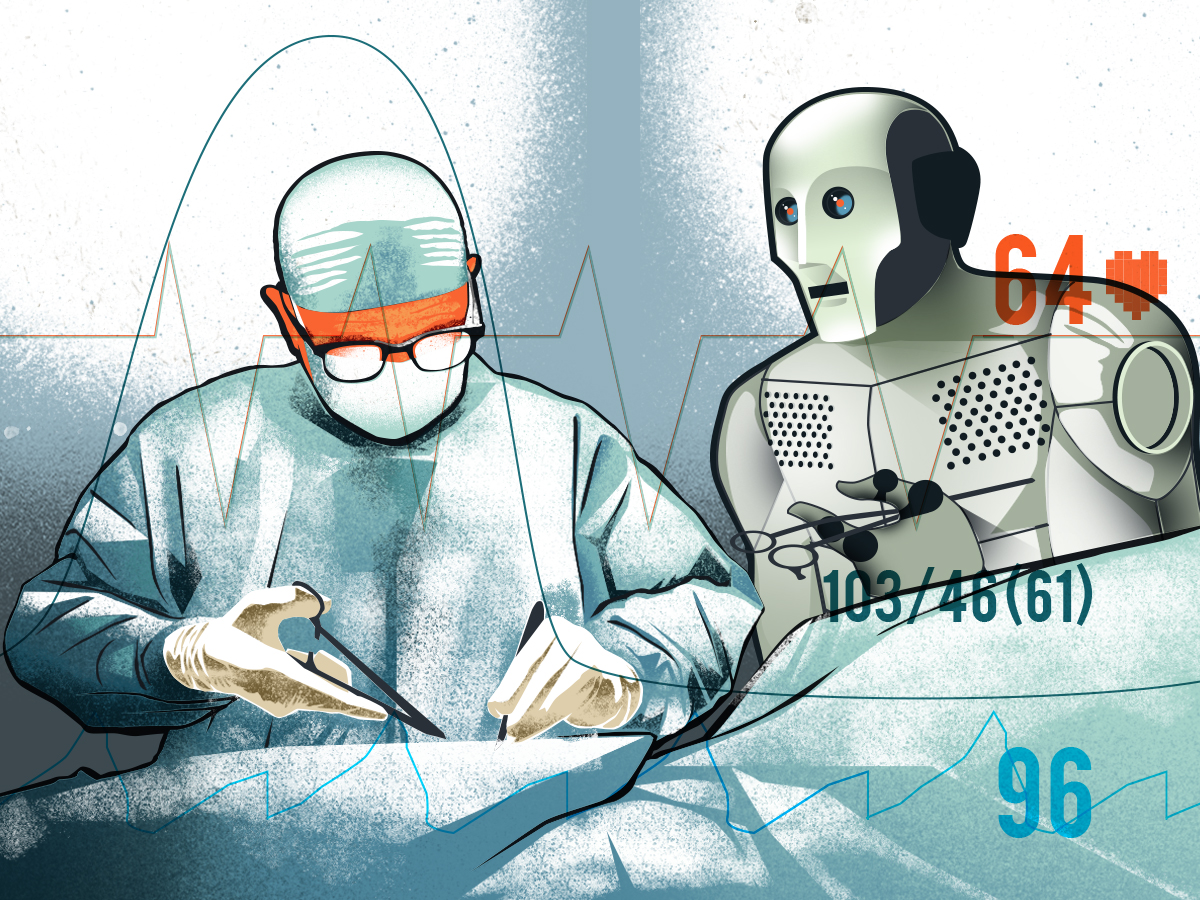The image is a detailed graphic design, possibly created by a computer, depicting a surgeon in the midst of performing surgery. The scene is reminiscent of a cartoon with animated characters. The surgeon is wearing typical surgical attire: a blue surgical cap, blue surgical mask, a surgical gown, white rubber gloves, and black plastic frame glasses. The doctor is holding black forceps in the right hand and a scalpel in the left, seemingly making an incision on the patient.

Adjacent to the surgeon is a predominantly white robot, resembling a surgical nurse, which is handing or about to hand another pair of forceps to the doctor. This interaction underscores the growing role of AI in assisting with tasks traditionally performed by humans. Additionally, the image includes medical statistics such as a red number "64" with a heart symbol next to it, possibly indicating a heart rate, and a blue "96" at the bottom, providing another measurement. The overall composition of the image reflects the integration of technology and AI in medical procedures.